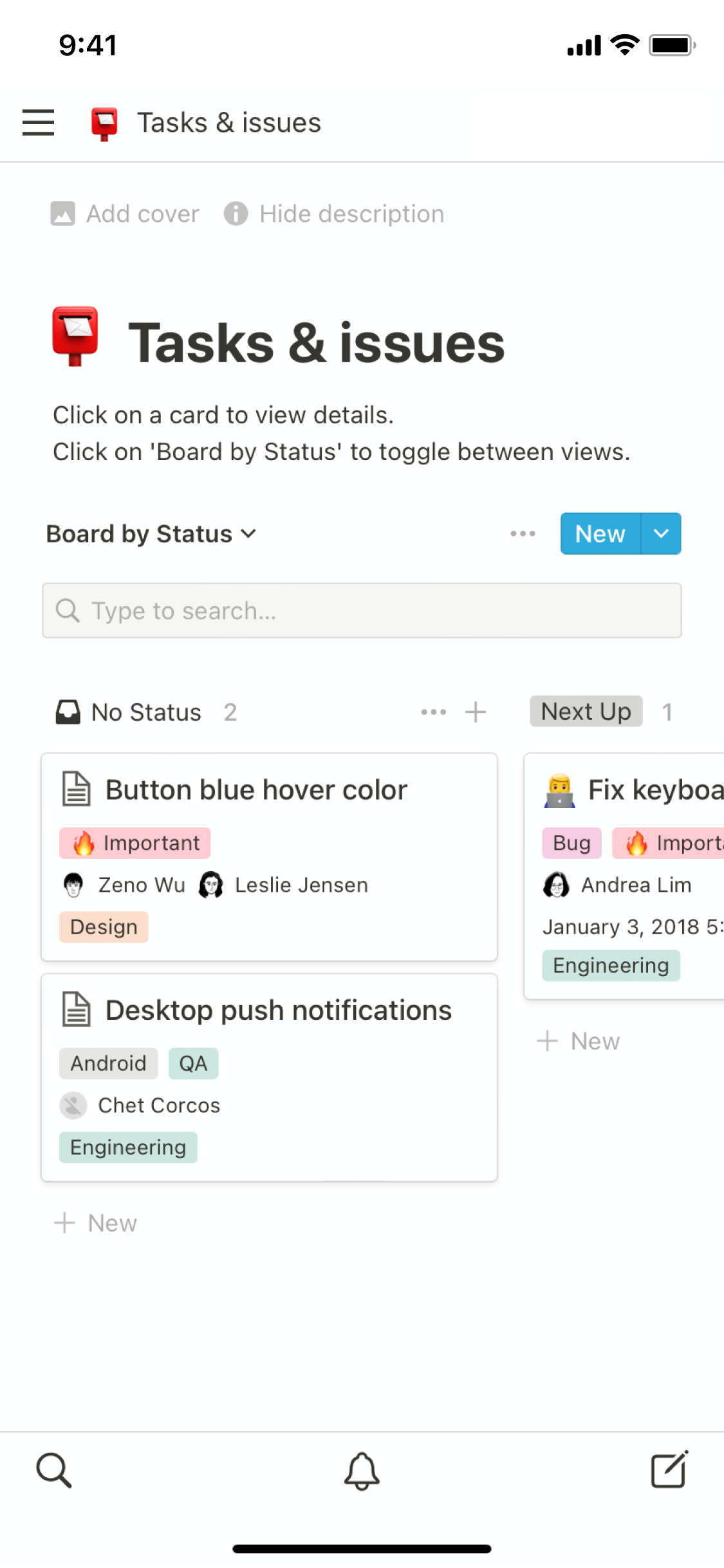The image is a screenshot from a cell phone. It is a vertical rectangle with a white background and black text. 

In the upper left corner, the time is displayed as 9:41. The upper right corner shows icons including the Wi-Fi symbol, battery indicator, and signal bars. Next to these icons, there is a small red word bubble containing a piece of paper, labeled "Tasks and Issues."

Further down, in bold text, it says "Tasks and Issues." Below this, instructions are given: "Click on a card to view details. Click on Board by Status to toggle between views." 

Following the instructions, the text "Board by Status" is displayed above a search bar. 

Below the search bar, there is a detailed area with different colored highlights indicating various categories. 

- "No Status" is displayed with a blue hover color.
- The word "Important," highlighted in pink, stands out prominently.
- The term "Design," highlighted in orange, is also visible.
- Another box contains "Desktop Push Notifications" with the category "Q and A" highlighted in green.
- The category "Engineering" is also highlighted in green.

To the right, another box lists "Fix Keyboard," with "Bug" and "Important" highlighted in pink, while "Engineering" is highlighted in green.

The screenshot effectively showcases a task management or productivity application, displaying various tasks and issues categorized by their status and priority.